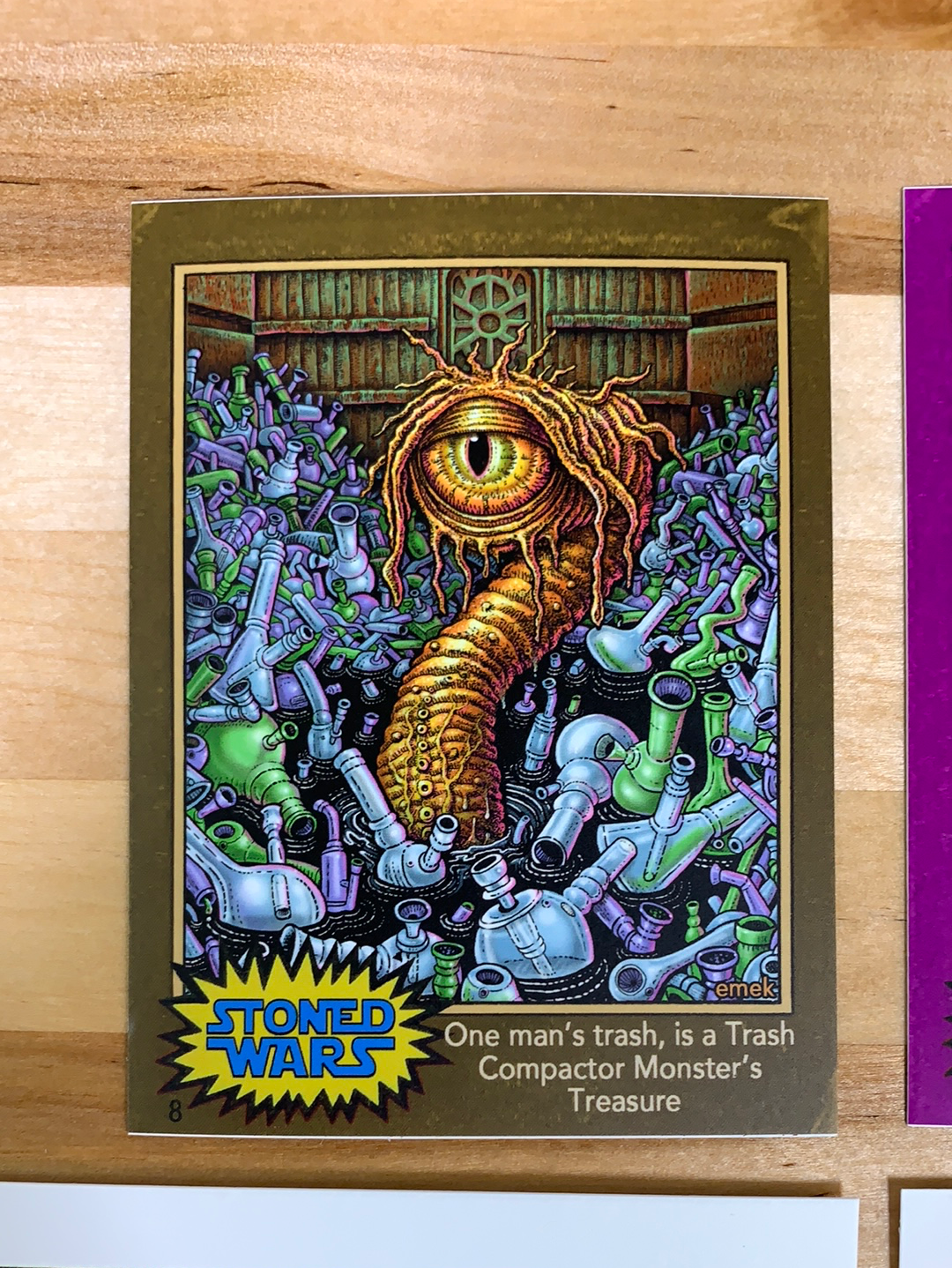The image depicts an illustration or poster mounted on a wooden wall composed of light sandy and light white planks. The central focus of the poster is a parody artwork that appears to be a play on Star Wars themes. It features a gold-colored, snake-like creature with a single large eye, surrounded by a chaotic assembly of bluish-green bongs of varying shapes and sizes, some of which appear to be floating in water. The background incorporates an intricate design with a teal circular pattern and lines. This snake-like creature also has vein-like appendages, giving it an organic, somewhat alien appearance. At the lower right portion of the poster, a jagged yellow circle with a black outline frames a caption. In blue font, it reads, "Stone Dwarfs," followed beneath by the subtitle, "One man's trash is a trash compactor monster's treasure." To the right of the main poster, another poster is partially visible, distinguished by a noticeable purple line running vertically. The poster is framed with a brown and light brown inner border, adding a final touch to its immersive design.